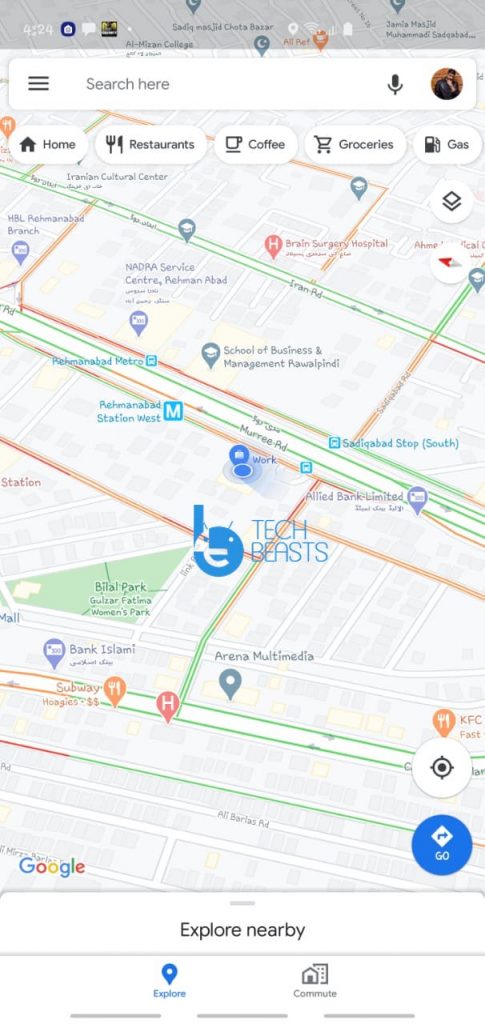This detailed map illustrates various key locations and amenities within a specified area. It features important places such as the Iranian Culture Center and the Brain Surgery Hospital, which is marked by a distinctive red circular icon with an 'H' inside. Other notable institutions include the School of Business Management, Ralpindi, identified by a teardrop-shaped logo adorned with a cap and gown symbol. 

Transportation options are clearly denoted, with the Rahamabad Station West metro station displayed as a square icon with an 'M'. There is also a blue circle that indicates a workplace location. 

The map highlights recreational areas such as Bilal Park, a women-only park represented by a triangle shape. For tech enthusiasts, the map shows the Tech Beasts location within a circle marked with a 'T'. 

Food and dining options are also well-represented, including a subway station with a fork and knife icon labeled "Hoagies," which comes with two dollar signs indicating moderate pricing, and a KFC in the lower right-hand corner. 

Additionally, the map features a user-friendly search box and an audio search function for ease of navigation. Directional assistance is provided with a blue circle icon that contains a diamond and an arrow pointing up and to the right.